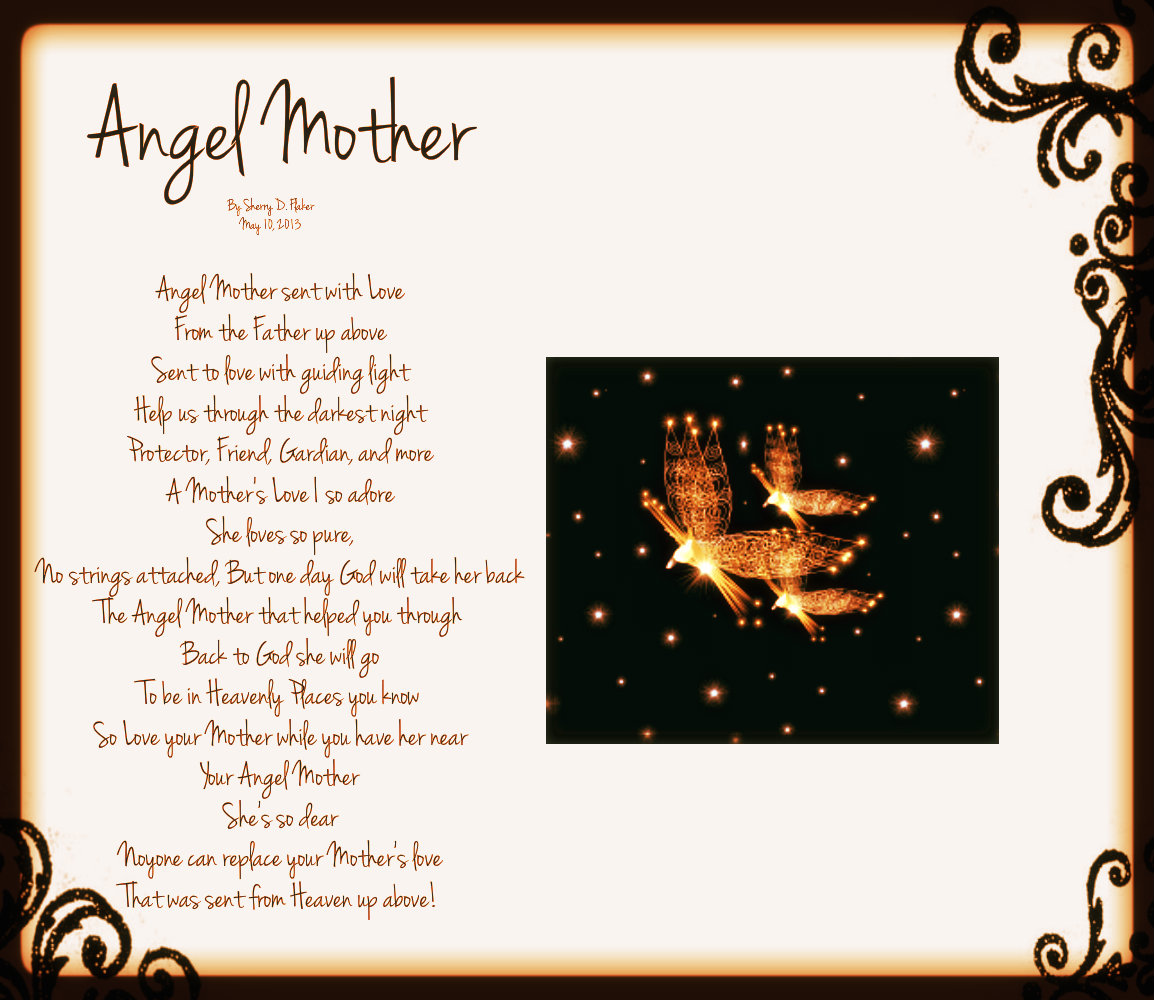The image is a square graphic design framed with a black border. It features intricate, filigree-like swirls and floral designs in the corners—specifically, the top right, bottom right, and bottom left, leaving the upper left corner plain. The central background of the design showcases hues of black and orange with some subtle beige and glowy brown edges.

In the upper left corner, the title "Angel Mother" is written in large, black, seemingly handwritten text. Below this title, in smaller gold text, it reads "By Sherry D. Flaker" alongside the date May 10, 2013. The main body of the image contains a heartfelt poem in a brown or black gold typeface. The poem starts with "Angel Mother sent with love from the Father up above," and goes on to describe the guidance and pure love of a mother, who is depicted as a guardian and friend. The text emphasizes cherishing a mother's presence and acknowledges that her love is irreplaceable, sent from heaven.

Additionally, the design includes graphics of glowing fairies or doves and little stars or lights spread throughout, enhancing the celestial and emotive atmosphere of the piece.